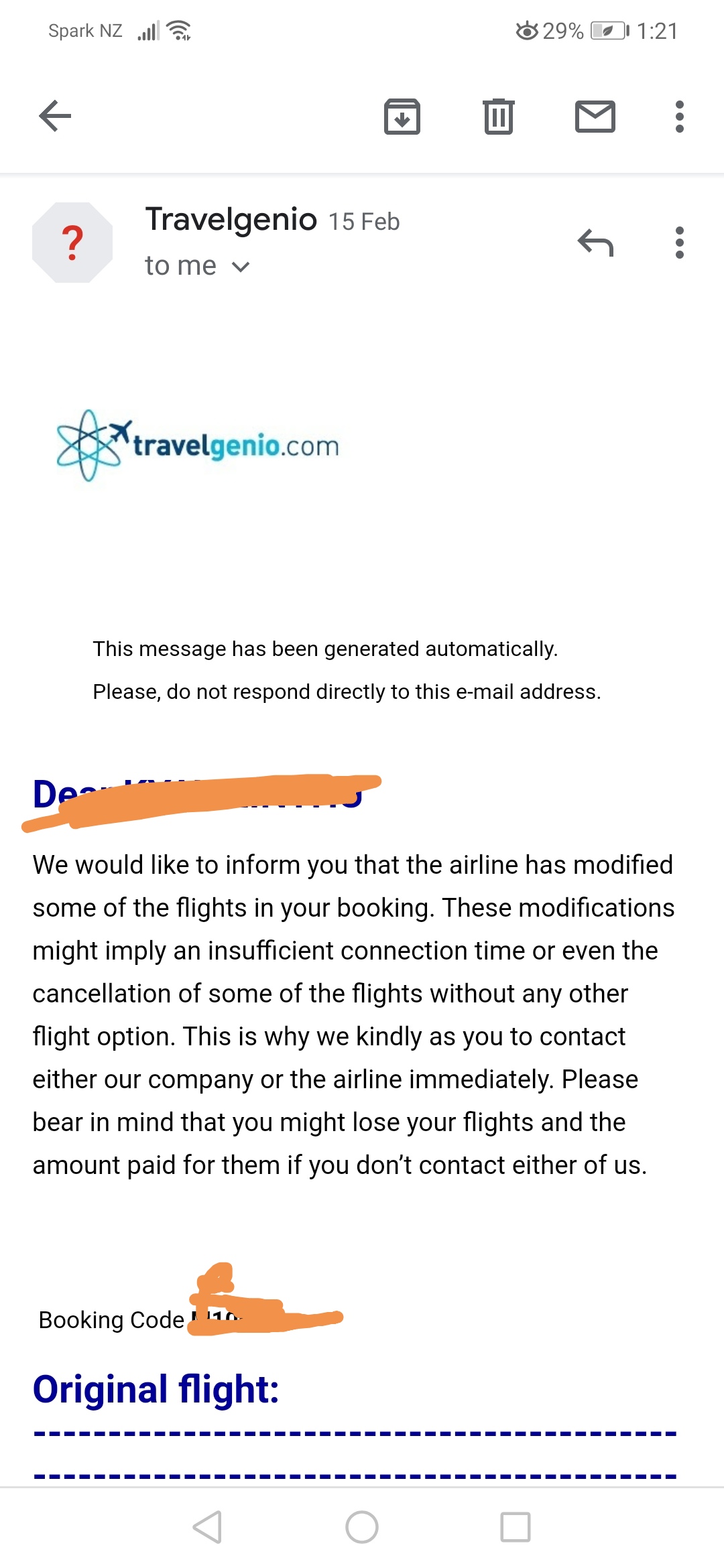The screenshot from an Android phone captures the device's status bar at the top, showing "Spark NZ" as the carrier with full cellular data bars, connected Wi-Fi, a 29% battery level, and the time as 1:21. Below the status bar, an email app is open, displaying an email from TravelGenio. The email's subject is about a modification in flight details. The sender warns that changes to the flight schedule may result in insufficient connection time or even cancellations without alternative options. The email urges the recipient to contact either TravelGenio or the airline immediately to avoid losing their flights and the money paid for them. It includes a booking code and details about the original flight. The interface also features icons for deleting the email (trash icon) and other email-related functions (envelope icon).